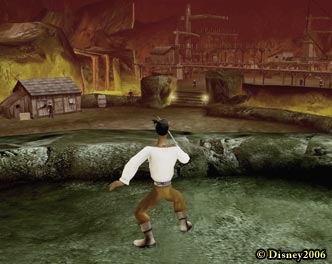The image appears to be a screenshot from an older, computer-generated video game, indicated by the Disney © 2006 watermark in the corner. The graphics suggest it may be a low-budget game from the time. In the foreground, a character dressed in a white long-sleeve shirt is visible, standing on the side with a sword in hand. The background features a small village, a pier, and a dimly lit scene that perhaps includes a smoldering or burning small city in the distance. The overall scene has a dark and somewhat ominous atmosphere.